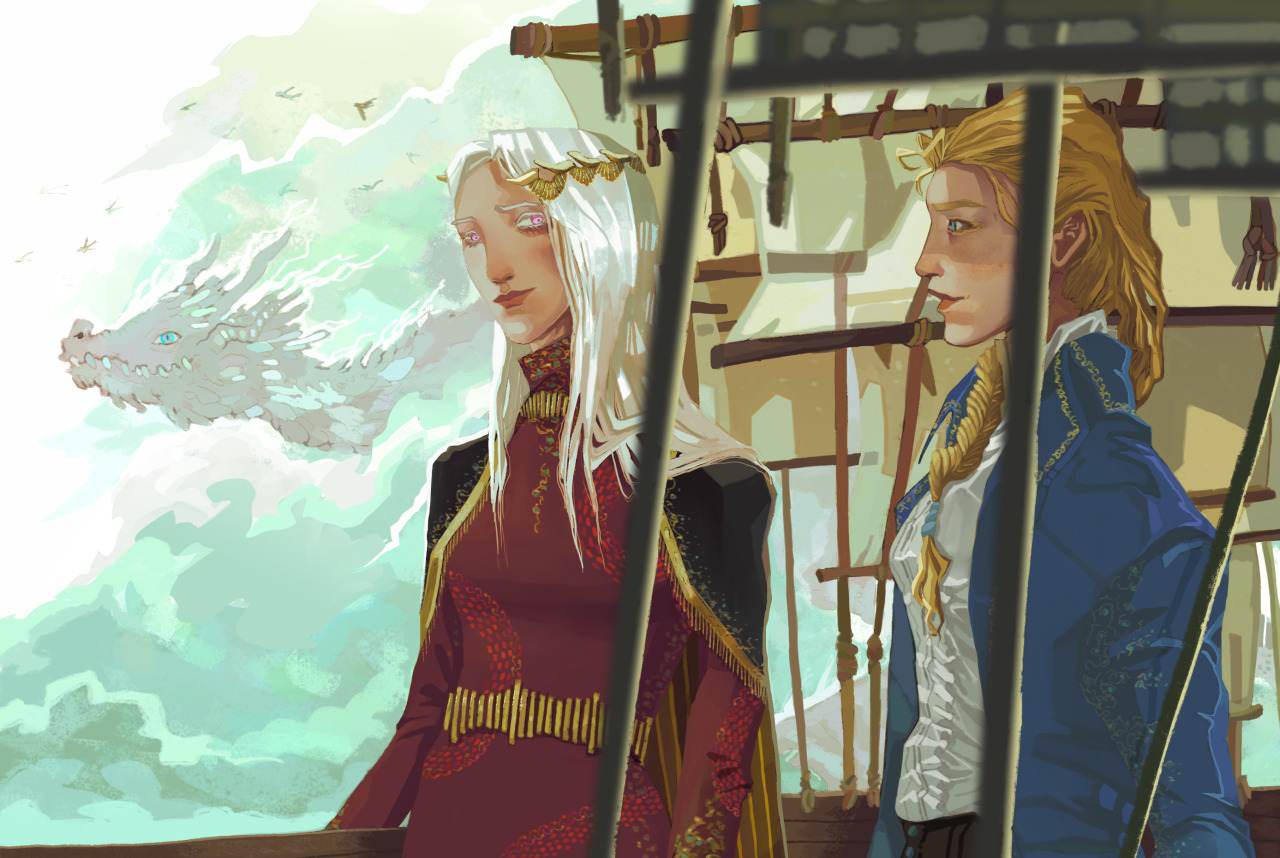This captivating painting portrays a young man and woman, evocative of the Renaissance period, standing on the deck of a ship with the abstract suggestion of sails overhead. The woman, with her long, silvery white-blonde hair, has her locks elegantly held in place by gold shell-shaped combs. She is dressed in a high-neck, form-fitting gown of deep wine color, adorned with an intricate red design. A black shawl drapes over her shoulders, complemented by a gold belt cinching her waist. 

The young man, gazing intently at the woman who looks wistfully into the distance, has long blonde hair styled into a voluminous braid. He is strikingly handsome, dressed in a royal blue jacket over a white ruffled shirt and collar, epitomizing Renaissance elegance.

The sky above them is tumultuous, painted with swirling clouds in various shades of gray, white, and pale seafoam green, suggesting an approaching storm. Amidst this dramatic backdrop, a spectral wolf's head with a bright blue eye and menacingly sharp teeth emerges from the clouds, adding an element of mysticism and foreboding to the scene.